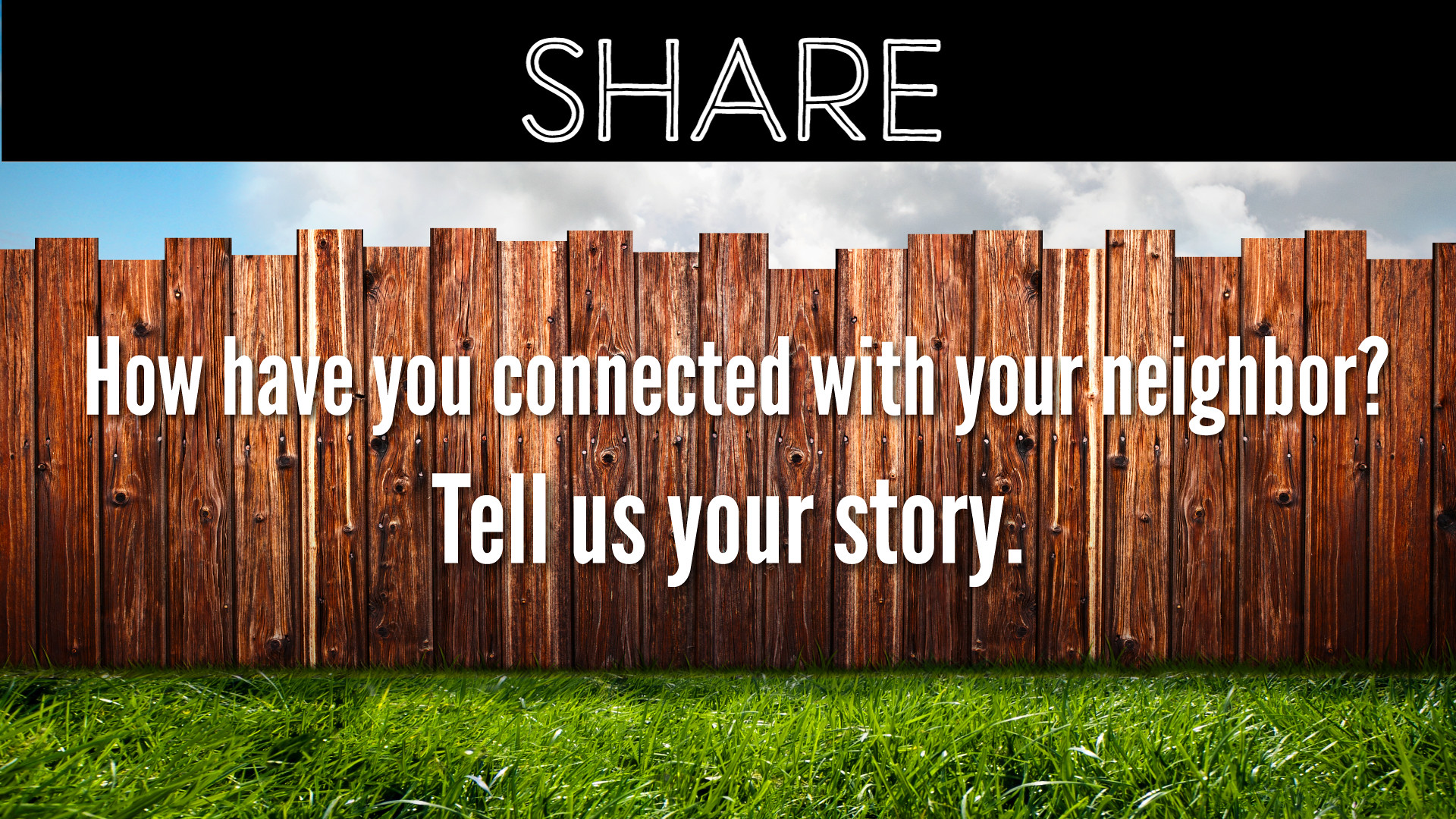The image displays an oblong-shaped poster divided into distinct horizontal sections. At the top, a thick black band spans across the width, featuring the word "SHARE" in prominent white letters with black filling the middle of the letters. Just beneath this strip, a thin sliver of blue sky stretches horizontally, scattered with white clouds. Dominating the center of the poster is a rustic wooden fence characterized by its irregular, differently sized slats and visible knots. This fence, rendered in shades of brown with occasional white spots, bears the white text: "How have you connected with your neighbor?" followed by a prompt in larger font, "Tell us your story." The fence is grounded by a lush expanse of green grass at the bottom, illuminated by sunlight and casting shadows on the fence. The overall composition and text suggest an invitation for people to share their stories of connecting with neighbors, likely for a community project or website.